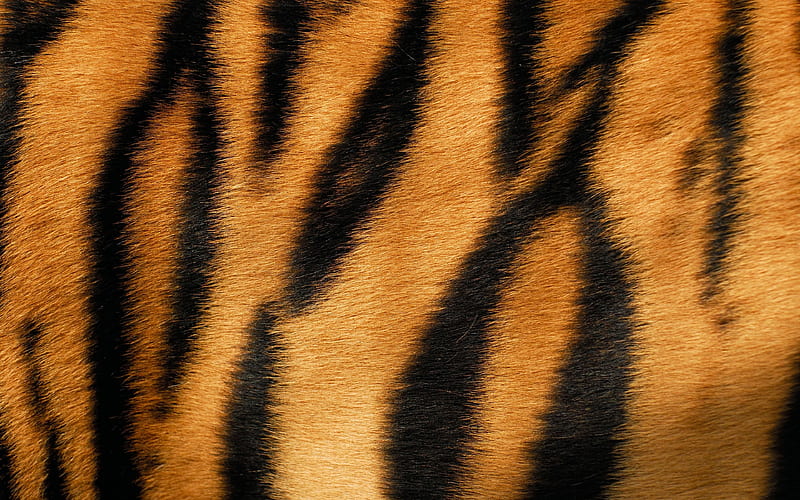This photograph captures an extreme close-up of what appears to be a tiger's fur, revealing its iconic pattern of black stripes set against a backdrop of vibrant orange or possibly tan fur, depending on the lighting. The detail in the image is remarkable, showcasing the texture and slickness of the fur. The stripes are asymmetrical, running in various directions but predominantly from top to bottom. They vary in shape and size; some are short and straight while others are longer with splits and oblong offshoots. The image is slightly blurry, adding to the ambiguity of whether we are observing an actual tiger's hide or a meticulously designed rug mimicking the animal's pattern. The lack of sharp edges in the pattern, combined with the absence of geometric shapes, suggests a natural rather than a manufactured texture.